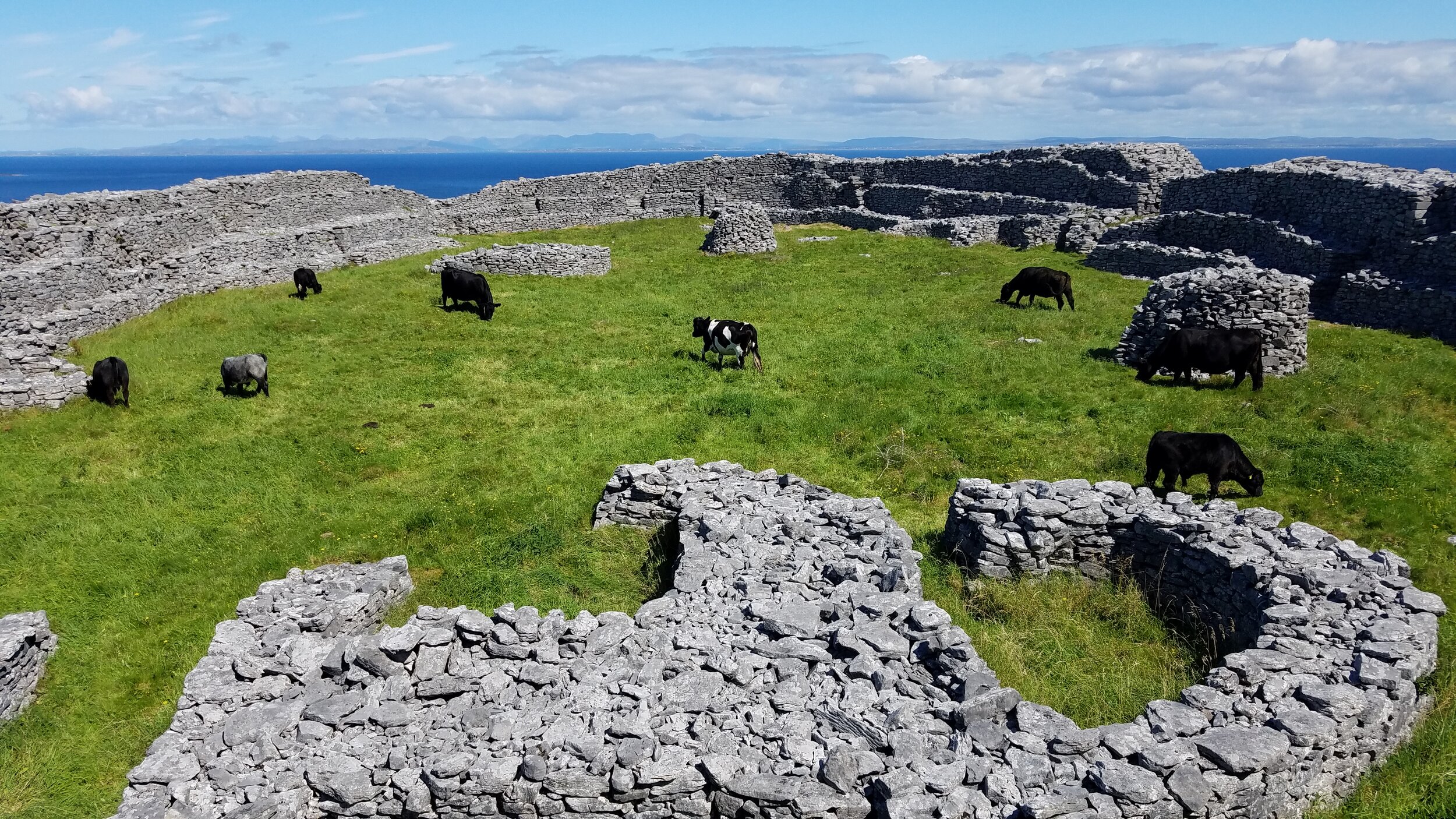In this color landscape photograph taken from a drone, the scene encompasses the serene countryside of either England or Ireland, bathed in a panoramic view that beautifully intertwines natural and historical elements. Central to the image are ancient multi-walled stone structures, their gray rocks meticulously arranged to form both complete and fragmented circular formations. These ruins, some as high as two to three stories, suggest a rich, albeit mysterious past. Enclosed by these stone walls, a lush green pasture serves as a grazing ground for a number of cows. The cows, predominantly black with a few black and white ones, dot the landscape, leisurely feeding on the vibrant grass.

In the foreground, the stone walls create intriguing shapes and patterns, including one that vaguely resembles a sideways face with an eye. Further back, more stone formations can be seen on the right side, adding depth to the historical ruins. The background is graced by the striking blue ocean, its calm presence harmonizing with the scene. Above, the sky is a clear blue adorned with light, wispy cumulus clouds, enhancing the tranquil and timeless quality of this pastoral setting.